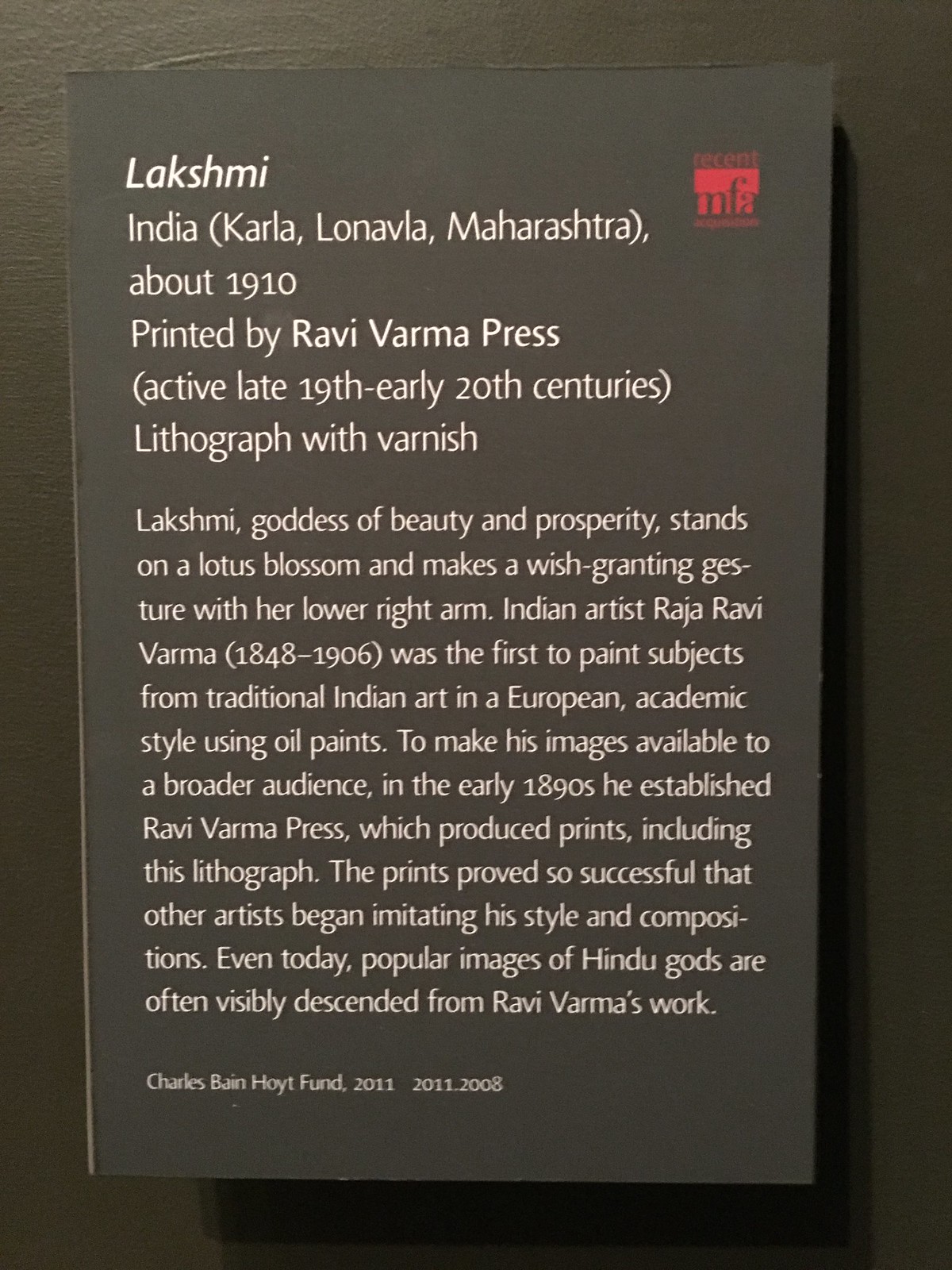This color photograph captures a descriptive plaque mounted on a dark gray wall within a museum display. The plaque, made of dark gray cardboard, details the artwork and legacy of the goddess Lakshmi. It features bold white text reading "Lakshmi" at the top, accompanied by a red square logo on the right that contains some illegible text. Below "Lakshmi," the plaque states "India, printed by Ravi Varma Press" with a date of 1910, and describes the artwork: Lakshmi, the goddess of beauty and prosperity, stands on a lotus blossom making a wish-granting gesture with her lower right arm. The text elaborates that Ravi Varma Press, established by Indian artist Raja Ravi Varma (1840-1906), was active in the late 19th and early 20th centuries, producing lithographs like this one to make traditional Indian art accessible to a broader audience. It notes that Ravi Varma's style has influenced depictions of Hindu gods ever since. At the bottom, in small white text, it acknowledges the "Charles Bain Hoyt Fund 2011-2008."